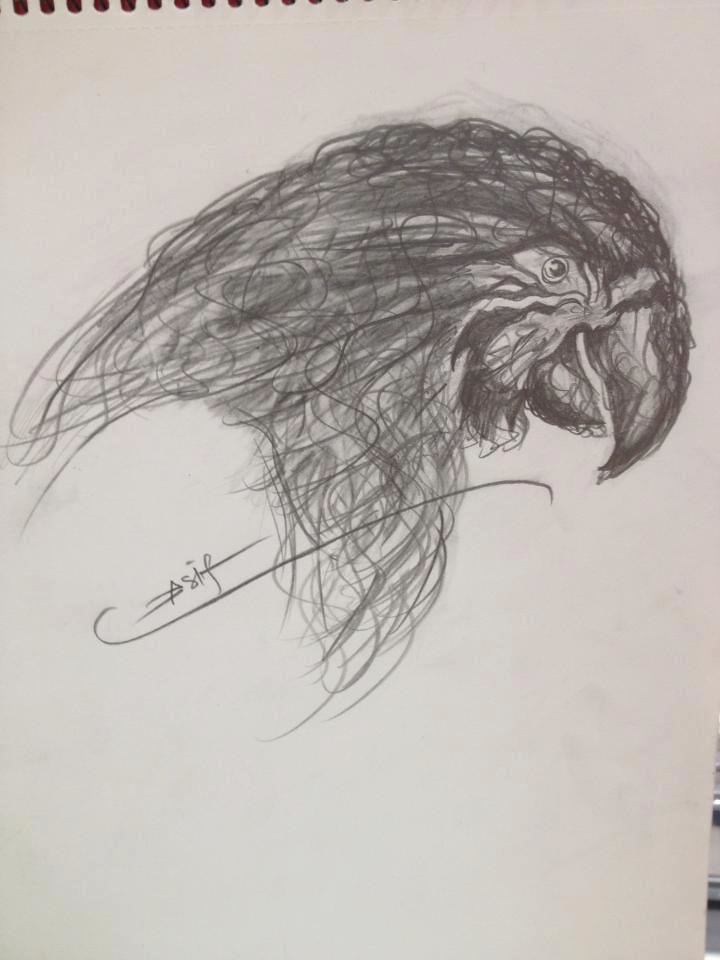This image captures a detailed pencil drawing of a parrot on a white sheet of paper torn from a sketch pad. The parrot is illustrated in profile, facing right. The artist has intricately depicted the parrot’s head, focusing on the facial features and the beak. The beak extends straight downward before tapering to a pointed tip directed leftward.

The feathers of the parrot are drawn with a combination of back-and-forth lines and circular squiggles, emphasizing the texture and the flow of the plumage. The artist has used curling lines to suggest the natural curvature of the feathers, giving the drawing a dynamic and lifelike appearance. At the bottom of the drawing is a small, elegant swoosh with the inscription "A-S-I-F," potentially the artist's signature.